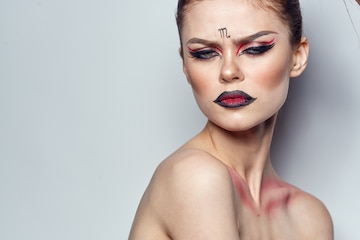This photograph, taken indoors against a light gray wall, features a woman of Caucasian descent from the shoulders up, with a focus on intricate face and body makeup. The woman faces right with her head turned over her right shoulder, her brown hair slicked back and partially cropped out of the frame. Bare-shouldered, she displays red paint above and below her clavicle. Her facial makeup is elaborate: heavy black eyelashes, dark pink eye shadow with red lines extending from the inner corners over her eyelids, making her eyes appear half-closed in an intense glare. Her eyebrows are elongated and narrow, and the letter M is painted between them, possibly evoking an astrological symbol such as Virgo. She sports dark red lipstick boldly outlined in black, giving her an angry pout. Her high cheekbones are accentuated by blush, contributing to her striking, somewhat angry appearance. Her makeup and the overall presentation suggest a dramatic, possibly conceptual or fashion-focused, look.